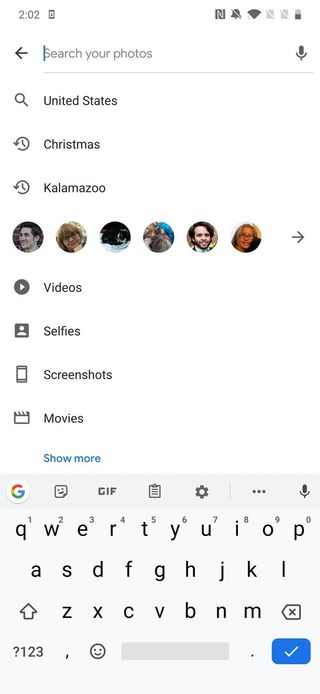The image shows a smartphone screen displaying a photo search interface. At the top left corner, there is a text field labeled "Search your photos," accompanied by a large button. Below this, in grey text, are sections titled "Recent Searches," which include the entries "Unlimited United States," "Christmas," and "Kalamazoo," each with a grey search icon on the left.

Further down, there are six slightly blurred profile images of people displayed horizontally. Below these profiles, a series of categories are listed, each with a corresponding grey icon on the left: "Videos," "Selfies," "Screenshots," and "Movies." The last item in this list is a blue "Show More" link, distinguishing itself from the otherwise black text on the white background.

At the bottom of the image, an open QWERTY keyboard is visible. This Google keyboard features a blue button with a white checkmark on the bottom right. The keyboard displays a "G" icon at the top left, with the "G" in Google's signature red, yellow, green, and blue colors within a white circle. Tabs for "Images," "GIF," "Paste," "Settings," "Menu," and "Mic" are located above the keyboard. The overall keyboard color is grey.